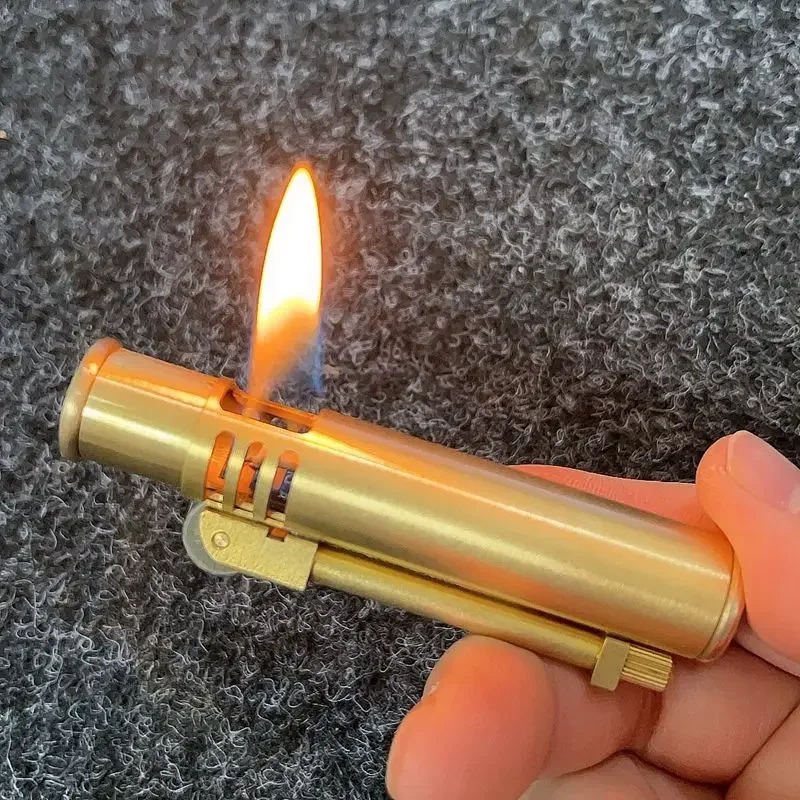The image depicts a close-up of a hand, likely belonging to a white person, holding a unique, cylindrical lighter with a golden or brass hue. The lighter, which has an unusual and vintage design reminiscent of old-fashioned cigarette lighters, features several openings: three small vents on the side and one larger hole on top, from which a small flame with a yellow tip and a blue base emerges. The hand is grasping the lighter with the thumb, middle finger, and index finger, which rests on the back of the tube. Additionally, a small brass latch is visible near the bottom, though it appears non-functional. The backdrop is a textured gray and black surface, possibly a fluffy, shag-like carpet with numerous curls, adding to the image's intricate detail.